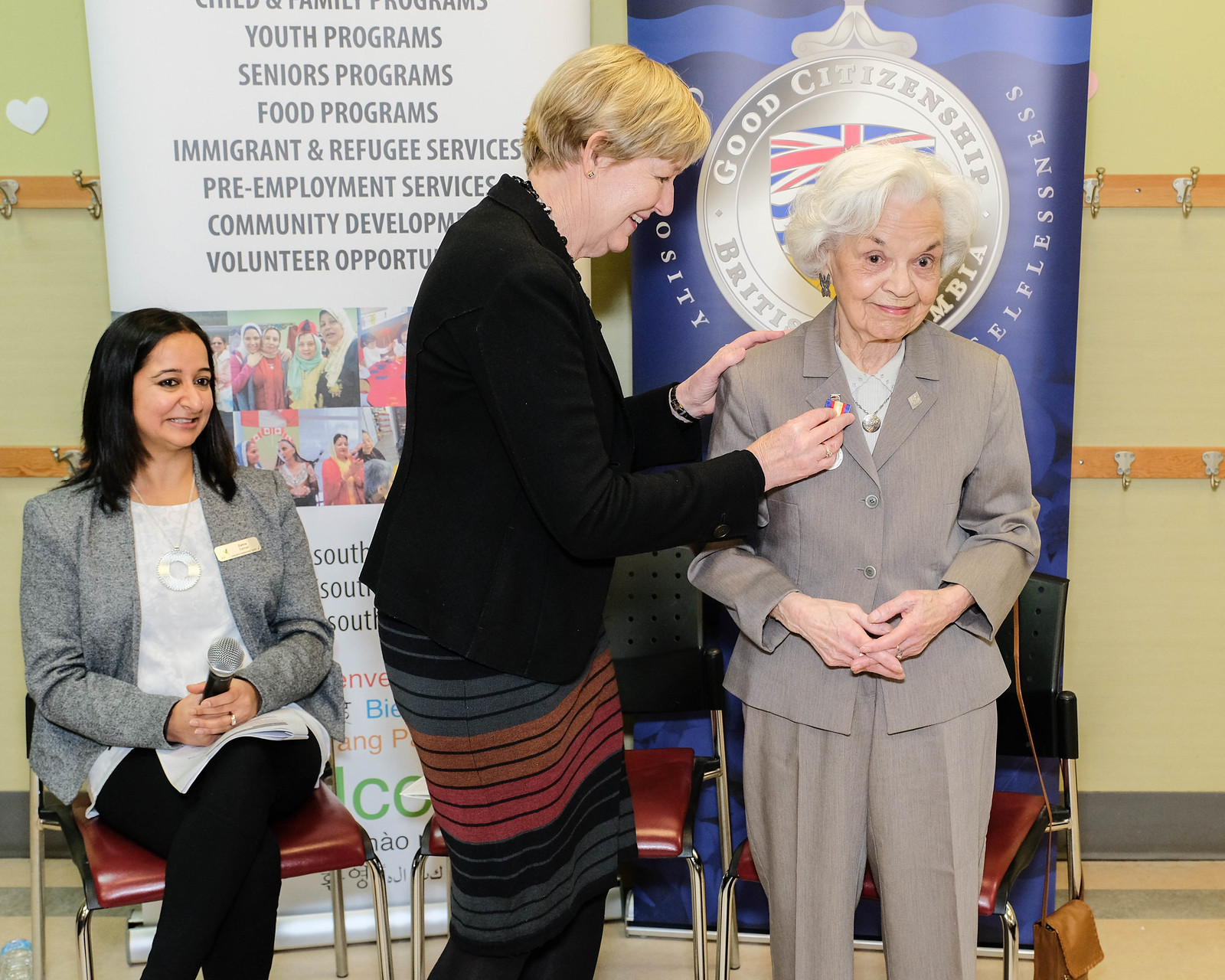In this detailed scene, a woman with short blonde hair, dressed in a black jacket and a horizontally striped skirt in black, red, orange, and gray, is seen pinning a medal onto the lapel of an elderly lady. The elderly lady, who appears to be in her 80s, is standing and wearing a gray suit. This interaction is part of a recognition ceremony, evidenced by the banner behind them, which lists various community services like youth programs, senior programs, school programs, immigrant and refugee services, re-employment services, and volunteer opportunities. Further in the background, a third woman with black hair, wearing a gray jacket and black pants, sits holding a microphone and smiling warmly at the sight of the award being pinned. Another prominent poster behind this third woman states, "Good Citizenship, British Columbia," with the Union Jack flag, underscoring that the event is honoring the elderly woman for her contributions to good citizenship. This touching moment captures the spirit of community appreciation and recognition.